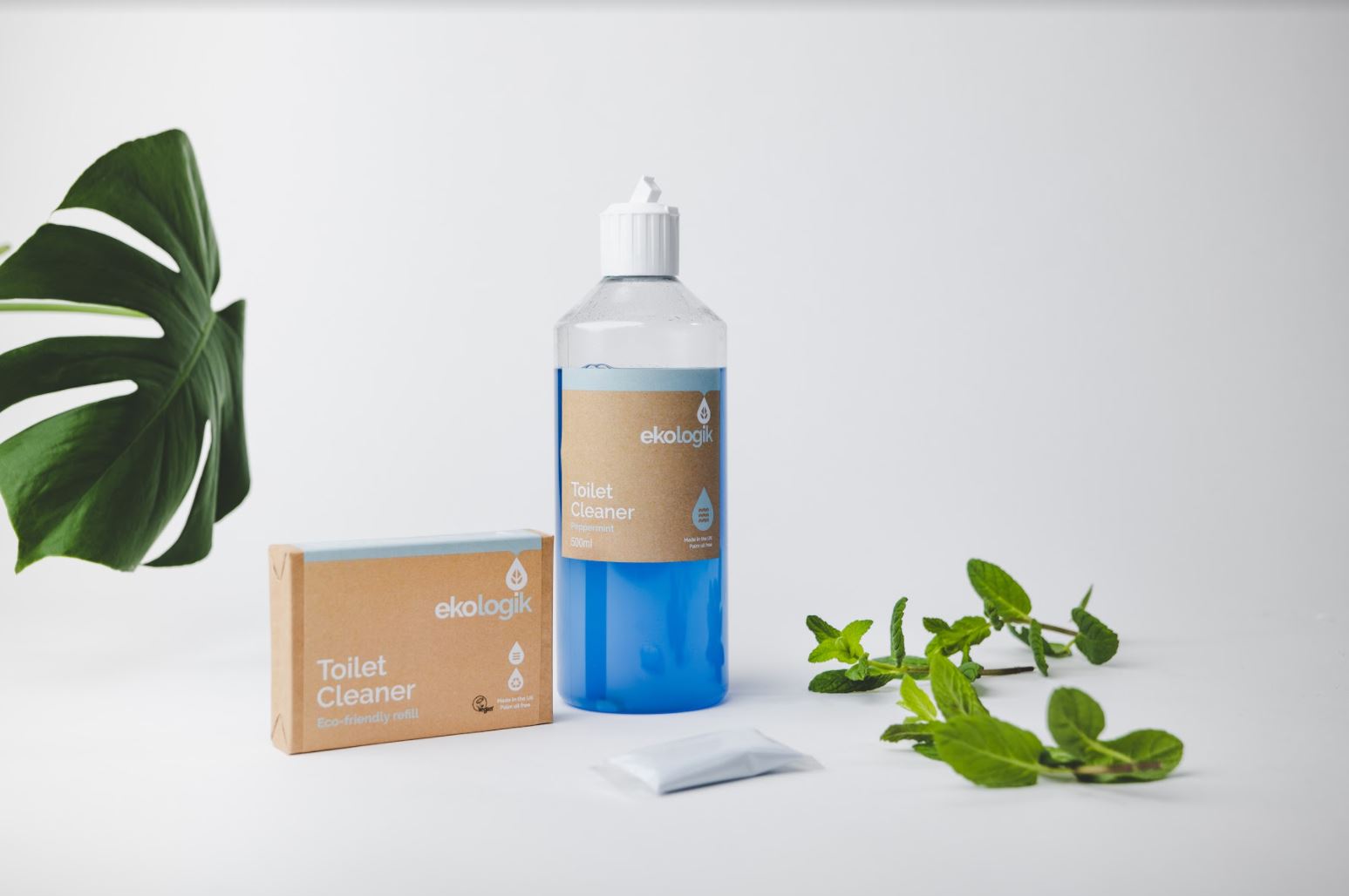In the photograph, a pristine white background serves as the canvas for an advertisement featuring Ecologic toilet cleaner products. Dominating the left side, there is a large, dark green leaf with distinct openings and a spine running through the middle, possibly AI-generated or digitally enhanced. In the center lies the focal point: a transparent plastic bottle filled with blue liquid, labeled "Ecologic" in white against a brown background, with a white squeezy cap. Accompanying the bottle, towards the left, is a brown cardboard box also labeled "Ecologic" and "Toilet Cleaner" in white lettering, with a small white sachet positioned in front of it. To the right of the bottle, small light green oval-shaped leaves, likely peppermint, rest delicately on the white surface, contributing a natural, fresh ambiance to the presentation.